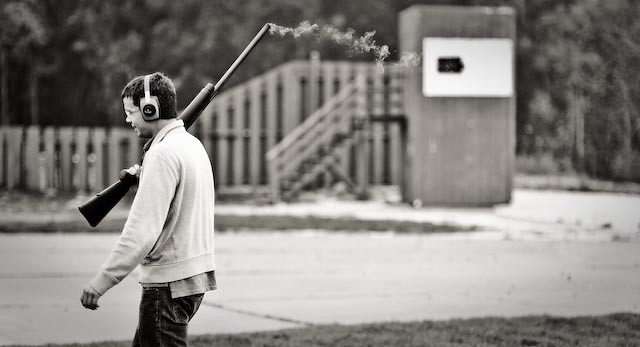In this landscape-oriented black-and-white photograph, a man's side profile is visible in the bottom left corner, walking towards the left. He appears to be in his 30s, with dark hair, glasses, and wearing noise-canceling headphones. He is dressed in a cardigan over a shirt and jeans, smiling as he holds a black shotgun, with smoke emanating from its barrel, suggesting it's just been fired.

The setting is outdoors, seemingly at a gun range, given the man's attire and the smoking gun. The ground in the image features a small patch of grass to the bottom right, a cemented area resembling a driveway or road in the center, and additional grassy areas in the background. There are various structures, including an observation deck, a staircase leading up to a building, and a fence. The distant background features a wooded area, adding depth to the scene. The entire image is rendered in shades of white, black, and gray, capturing a detailed and vivid moment in a serene, outdoor environment.